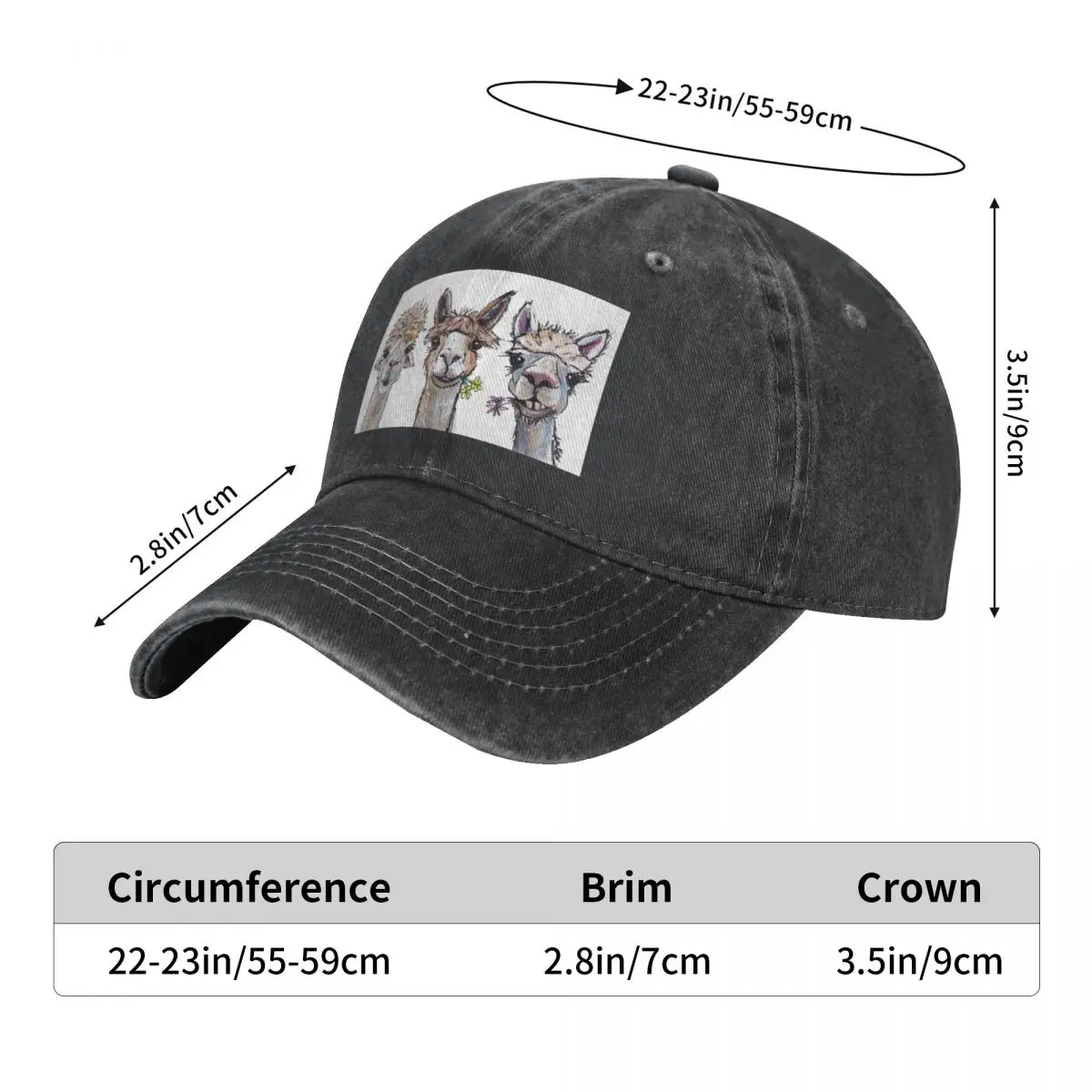This image is a detailed product listing for a black denim ball cap, set against a plain white background. The cap features a curved bill and is adorned with a white rectangular section on the front, showcasing caricature illustrations of three goats, each munching on grass. Detailed measurements are provided: the bill is marked as 2.8 inches (7 centimeters), indicated by a black arrow to the left. The top of the hat displays a circumference measurement of 22 to 23 inches (55 to 59 centimeters), while the height of the hat is noted as 3.5 inches (9 centimeters) on the right. Additionally, a gray box beneath the cap reiterates these dimensions in bold text labeled "circumference," "brim," and "crown."